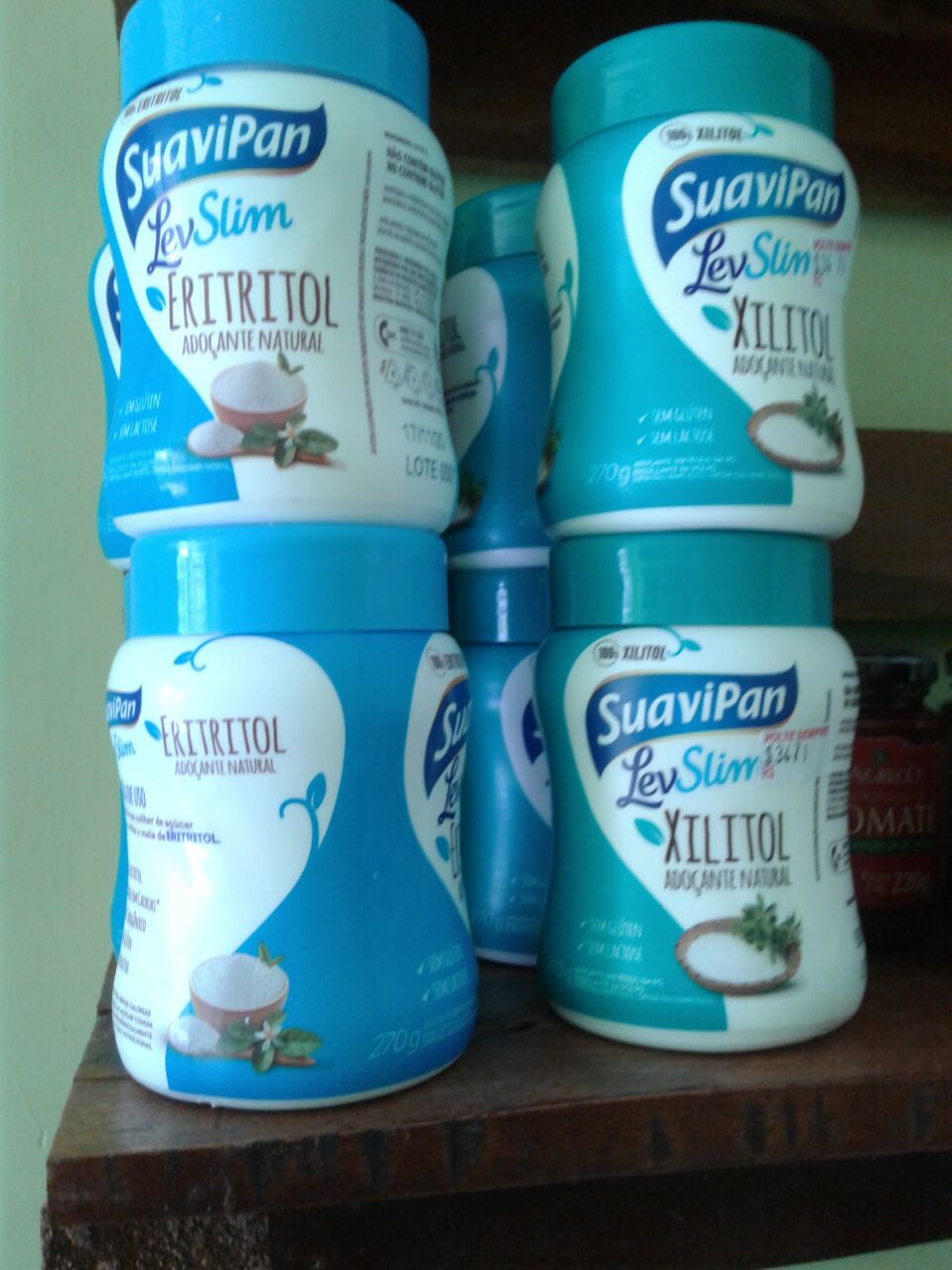The photograph captures a close-up view of several cylindrical containers displayed in a commercial setting. These containers, labeled under the brand "Suavipan," feature prominently positioned names and details. The containers are split into two distinct color schemes: the ones on the left are predominantly dark blue with white accents and dark blue lids, while the ones on the right sport a teal blue design with similar white accents and teal lids. The label showcases the text in a structured format: a dark blue ribbon with "Suavipan" in white text, followed by "Lev" in dark blue, and "Slim" in light blue. 

A price tag marked at $34.71 in white is also visible on the dark blue containers, which proclaim the product as Xanitol, with the word "natural" mentioned in a different language likely indicating its organic nature. The photograph is taken against a bluish-green wall backdrop, and the products appear to be stacked on a wooden surface, possibly implying a table or chair.

The arrangement includes four containers at the front, stacked two high, with additional containers partially visible behind them, suggesting a plentiful supply. The containers are more like short jars with wide screw tops rather than bottles. The two color variations might indicate different product types or flavors, with the dark blue ones possibly depicted with an image of yogurt and labeled "Erythritol," and the teal ones termed "Elexitol." Overall, the image emphasizes the uniformity and branding of the Suavipan products, highlighting their sleek design and stacked presentation.